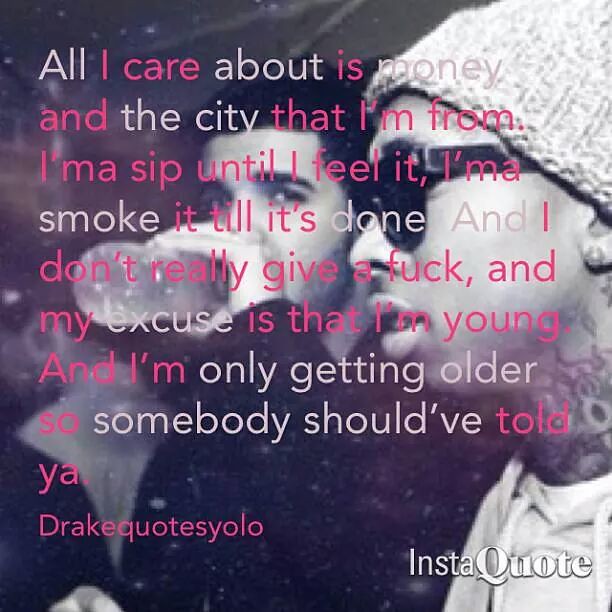The poster displays a black-and-white image of two young men. The first man, wearing sunglasses and a cap, has tattoos on his neck and a white sweatshirt. The second man, next to him, is captured drinking water while sporting a blue jacket. Dominating the image in large white and pink letters is a quote that reads: "All I care about is money and the city that I’m from. I’ma sip until I feel it. I’ma smoke it till it’s done and I don’t really give a fuck. And my excuse is that I’m young and I’m only getting older. So somebody should have told you." The attribution "Drake quotes YOLO" is emphasized in pink, while "insta quote" appears in white on the lower left corner. This scene could suggest a youthful Drake, with the overlay of his lyrics enhancing the imagery.